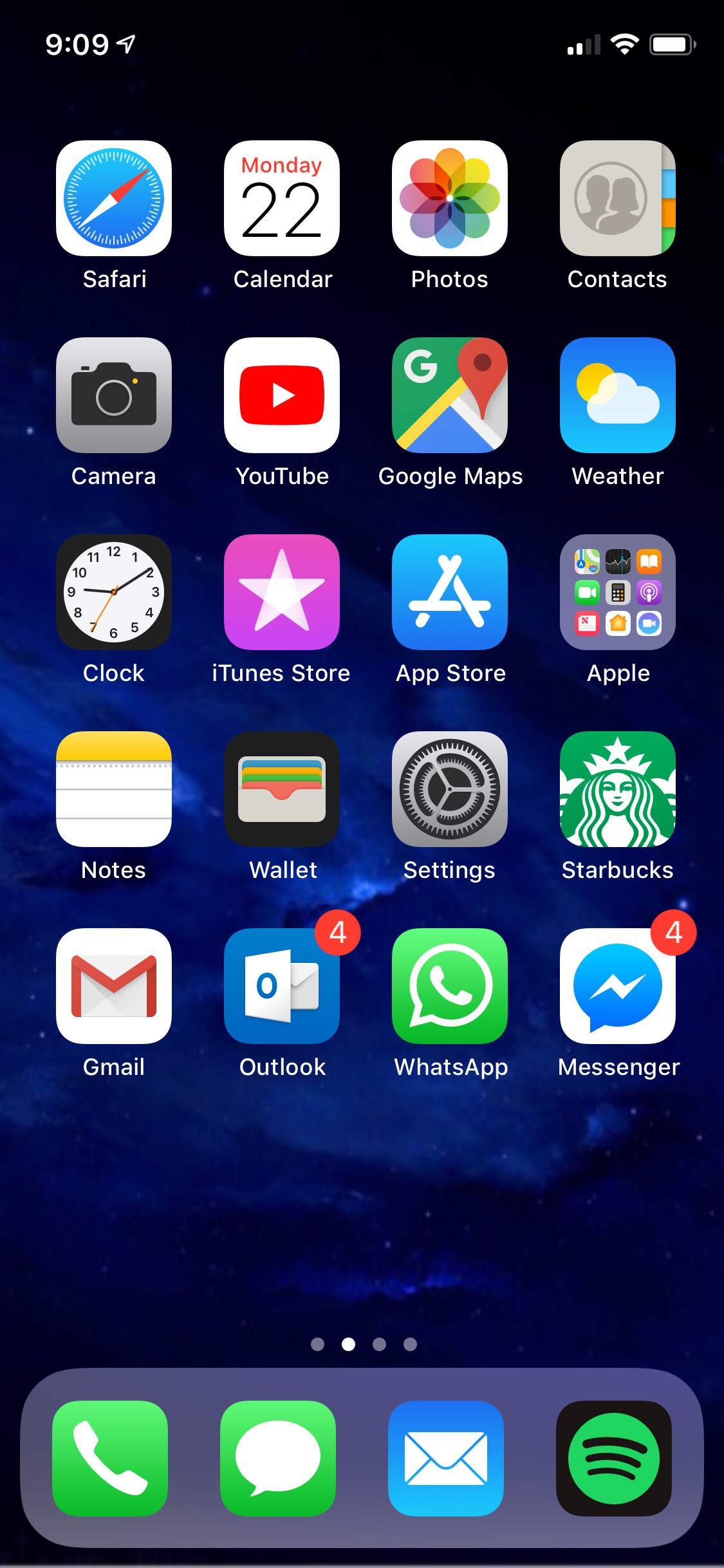This image depicts an iPhone home screen, likely from the 2010s, with a 5x4 grid layout for the app icons. The background image features a dark, heavily clouded sky, casting a deep blue hue over the screen. At the top of the display, the status bar shows the time at 9:09, location services activated, two bars of cellular signal, full Wi-Fi connectivity, and a nearly full battery icon.

At the bottom of the screen, the dock holds four frequently used apps: Phone, Messages, Mail (in blue), and Spotify (with its recognizable green circle on a black background). The main section of the home screen showcases a mix of standard and additional apps such as Safari, Calendar, Photos, and Contacts. Notably, the screen also includes non-default apps like Starbucks, Outlook, and Facebook Messenger. Both Outlook and Facebook Messenger have red notification badges, each displaying four unread notifications.

The user appears to be on the second of four available home screens, as indicated by the page dots at the bottom.